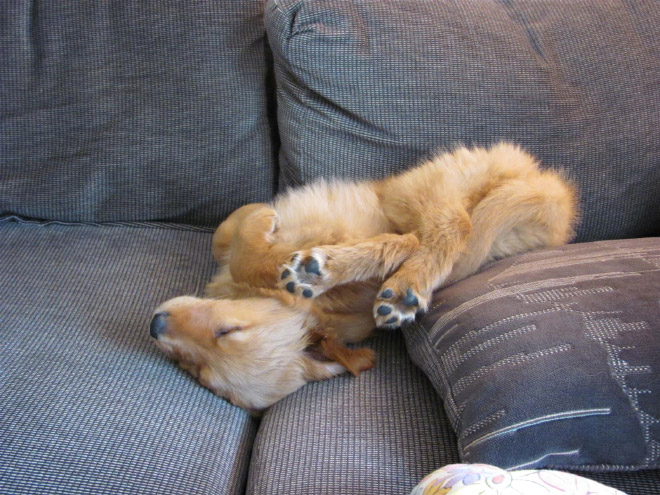In the center of this image is an adorable brown puppy, likely a golden retriever, peacefully sleeping on a plush gray couch. The couch appears to be made of a cotton-like fabric and shows a slightly blue tint, adding to its cozy feel. The back cushions are fluffy, and one cushion is solid gray with white markings resembling a cityscape, while the other has a mix of patterns. A slightly worn, dark gray pillow with a light gray design supports the puppy's rear end. The puppy is lying upside down with its head toward the left side and its feet sticking up in the air. Its head rests in the separator between the couch cushions, and one ear flopped behind its head. The puppy's little black nose and closed eyes exude a sense of pure contentment. Its front paws are curled up adorably at its chest, and its back legs are contorted sideways, showing the bottoms of its paws with black markings. Additionally, a white blanket with colorful flowers can be seen trailing off the edge of the image, enhancing the cozy atmosphere. The dog is the main focal point of the picture, radiating peace and happiness.